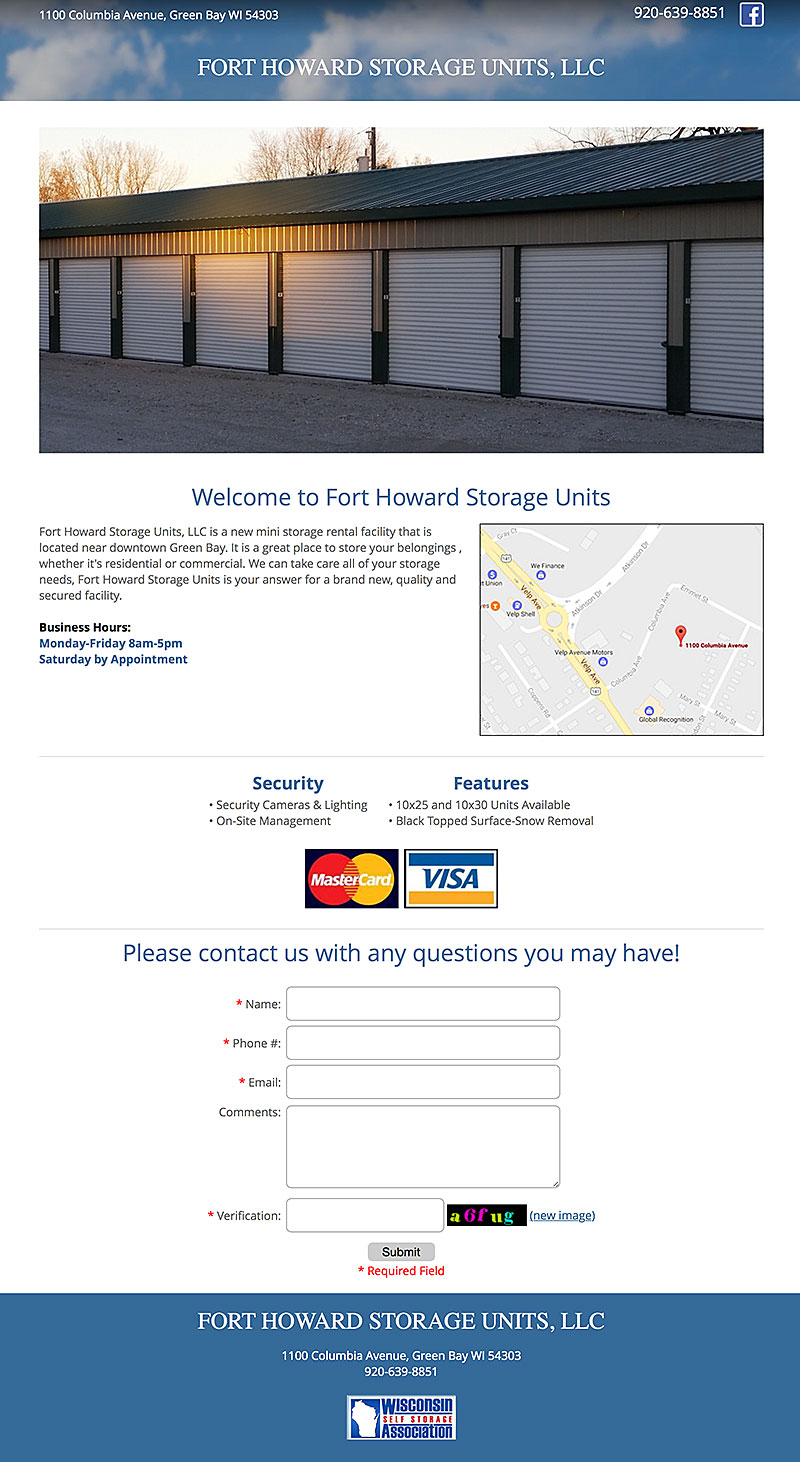The photo captures a page visible on someone's phone, displaying the details of Fort Howard Storage Units, LLC. In the upper left-hand corner, the address is clearly listed as 1100 Columbia Avenue, Green Bay, Wisconsin 54303. In the top right-hand corner, the phone number 920-639-8851 is prominently visible, alongside the recognizable Facebook logo, featuring a white "F" in a blue box.

The middle section of the page displays an image of the storage facility, which resembles a pole barn divided into multiple segments, each equipped with its own white garage door. Directly below the image, bold text welcomes readers to Fort Howard Storage Units.

The caption continues, explaining that Fort Howard Storage Units, LLC, is a newly established mini storage facility conveniently located near downtown Green Bay. It emphasizes the versatility of the units, suitable for both residential and commercial storage needs, highlighting the facility's modernity, quality, and security.

Further details include the company's business hours, a location map, payment options (accepting MasterCard and Visa), and additional finishing areas at the bottom of the page, providing a comprehensive overview of the storage unit services offered.